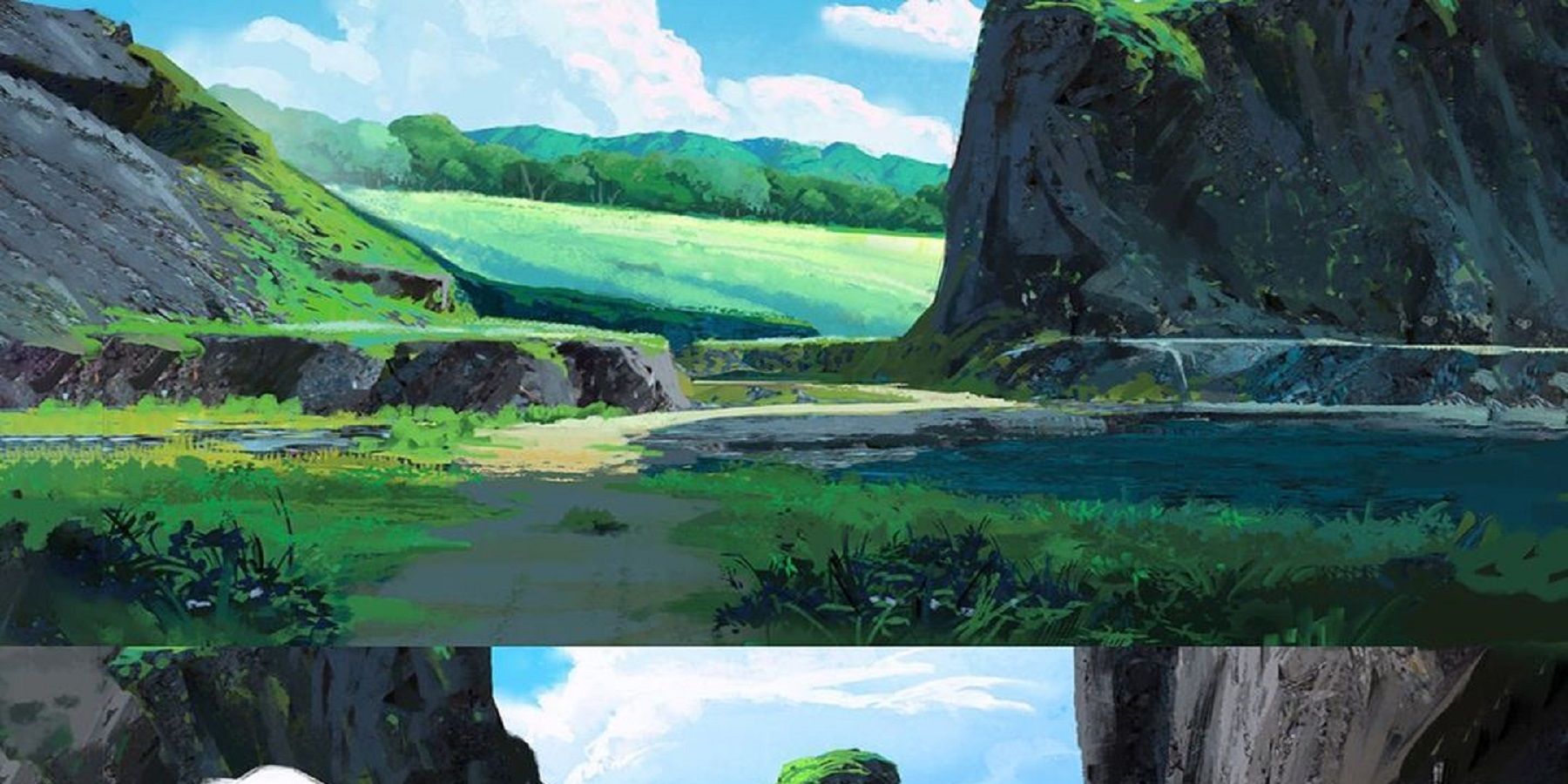The image is a nearly photorealistic acrylic painting that likely depicts a scenic UK landscape. Dominating the foreground are two expansive stone areas composed of medium to dark gray basalt rock outcrops. The left outcrop features a sloping surface adorned with green moss or grass, while the right outcrop appears more barren, with a lone tree emerging from it. Nestled between these rocky formations is a body of water, possibly a lake or stream, reflecting an upside-down image of the stones and sky. The reflective water also reveals grassy areas and small puddles of water scattered around the rocks.

In the middle ground, an open field of light green stretches out, bordered by a row of lush green trees. The far background is adorned with a vivid blue sky populated by large, white, fluffy clouds. The entire scene is rendered in a condensed color palette, featuring shades of gray, green, blue, and white, enhancing its visual cohesion. The overall composition captures a tranquil, natural setting with rolling hills and subtle vegetative growth, making it a serene and detailed portrayal of the landscape.